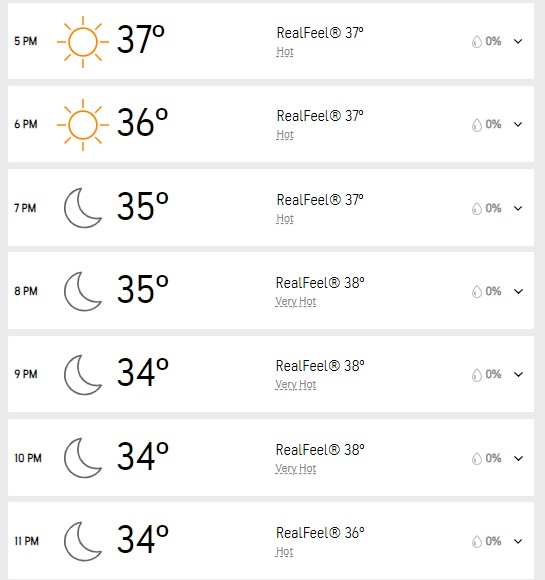The image presents a web listing displaying hourly weather updates with specific times and temperatures. The background is white, with black lettering and numbers conveying the information. 

- At 5 p.m., the forecast shows a sunshine icon, a temperature of 37 degrees, a real feel of 37 degrees, marked as "hot," and 0% precipitation. There is a clickable symbol next to the details.
 
- At 6 p.m., the display is similar with a sunshine icon, a temperature of 36 degrees, a real feel of 37 degrees, labeled "hot," and 0% precipitation. This line also has a clickable symbol.

- For 7 p.m., the icon changes to a partial moon, with a temperature of 35 degrees, a real feel of 37 degrees, described as "hot," and 0% precipitation.

- By 8 p.m., the icon shows a half moon, with the temperature remaining at 35 degrees, a real feel of 38 degrees, and still 0% precipitation.

- At 9 p.m., the half moon icon remains, but the temperature drops slightly to 34 degrees, with a real feel of 38 degrees, described as "very hot," and 0% precipitation.

- At 10 p.m., the forecast mirrors the previous hour, featuring the half moon icon, 34 degrees, a real feel of 38 degrees, "very hot," and 0% precipitation.

- Finally, at 11 p.m., the temperature stays at 34 degrees, with a real feel of 36 degrees, noted as "hot," and 0% precipitation.

Each hourly forecast includes a clickable link symbol for further details.